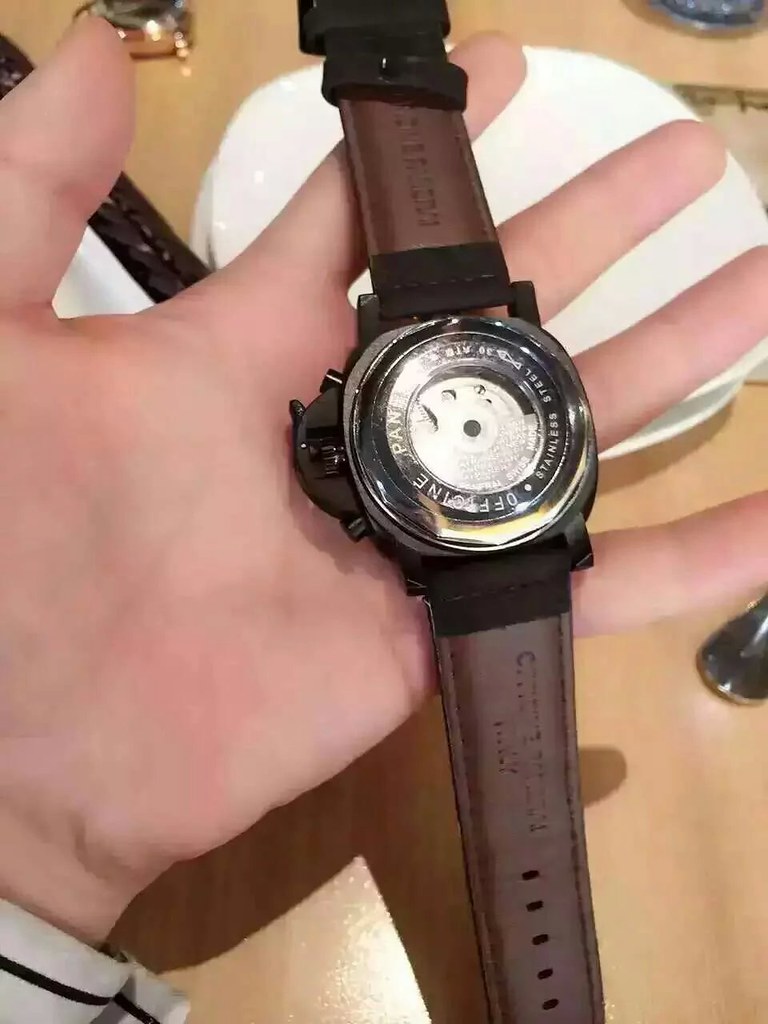This detailed photograph captures a man's outstretched hand, palm up with fingers spread, holding an upside-down Citizen watch. The watch features a deep brown leather strap and a stainless steel case with a black housing around the edges. Through a clear circular window on the back, you can see the intricate self-winding gears, showcasing its skeleton design. The watch, seemingly a prototype, lacks hands on its clock face which is turned face down. On the left side of the case are various dials and push buttons, with the main dial in the center protected by a half-dome metal piece. The man is dressed in a white shirt with black embellishments visible around the cuff. The background shows a light-colored dining table with a peachy hue, adorned with other watches, white bowls, and possibly china plates, emphasizing a smooth and possibly filtered aesthetic. The image appears meticulously arranged, suggesting a thoughtful and poised presentation.